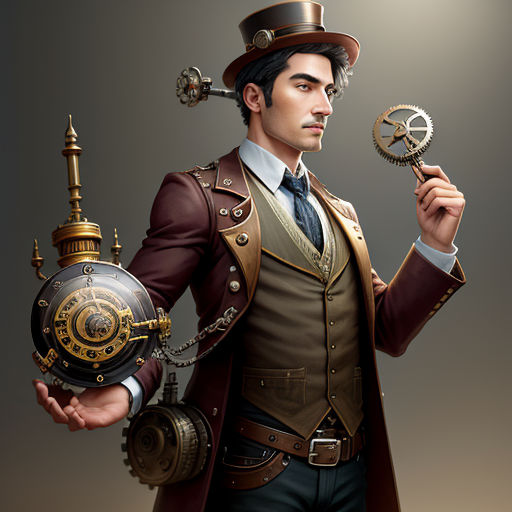This AI-generated image, resembling Joe Jonas as a steampunk doctor, features a highly detailed and intricate portrayal of a man with a blend of human and mechanical elements. He has dark brown hair, a slight mustache, and is wearing a distinctive top hat adorned with a silver clip and a pocket watch. His attire includes a white dress shirt with a navy blue tie, a medium brown vest trimmed in gold, and a dark brown, burgundy-toned leather jacket that appears almost wooden or metallic. He is adorned with multiple belts and dark pants, fitting the steampunk theme.

A monocle enhances his face, and a peculiar valve-like object protrudes from the back of his head. This character's right arm, extended outward, displays a clock-like device connected to his jacket by chains, while his left hand raises a wand-like stick topped with a gear. Notably, he possesses six fingers on his left hand. Additional accessories include a metal, gear-shaped canteen attached to his holster. The overall smoothness and minor inconsistencies in the depiction suggest AI generation, capturing the essence of steampunk aesthetics with an imaginative and otherworldly twist.